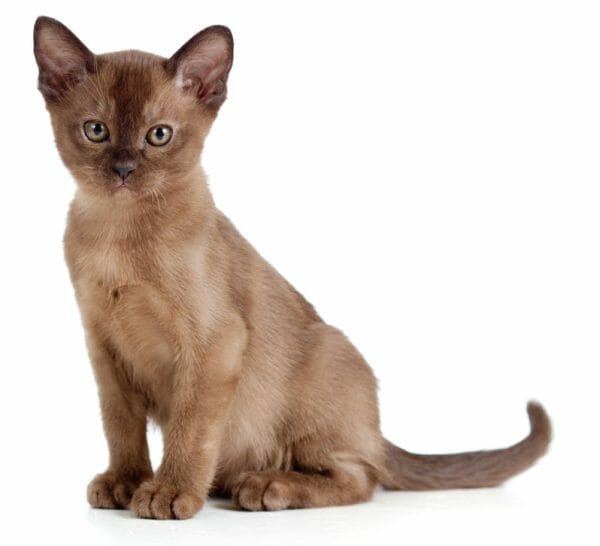This image presents a young kitten, predominantly light grayish-white with an intricate mix of shades accentuating its features. The backdrop is a stark, pure white, emphasizing the kitten's delicate hues. The kitten is positioned upright, gazing directly into the camera, its inquisitive expression captivating the viewer. Its slender frame and soft, fur-covered paws, devoid of visible claws, add to its gentle appearance.

The kitten's ears are perked up, with pink interiors contrasting against its fur. A notable dark gray streak runs from the top of its forehead, between its bright light green eyes circled by black, down to its black nose. Its white whiskers and eyebrows stand out against the face's delicate tones. The kitten's tail, slightly darker than the rest of its body, curls up at the tip, adding a playful touch to its poised stance.

Additional brownish shades and darker streaks throughout its fur, particularly on its tail and the sides of its slender body, offer a more intricate texture to its light coat. The kitten remains the sole subject of the image, standing as a portrait of youthful curiosity and subtle beauty against the minimalist backdrop.